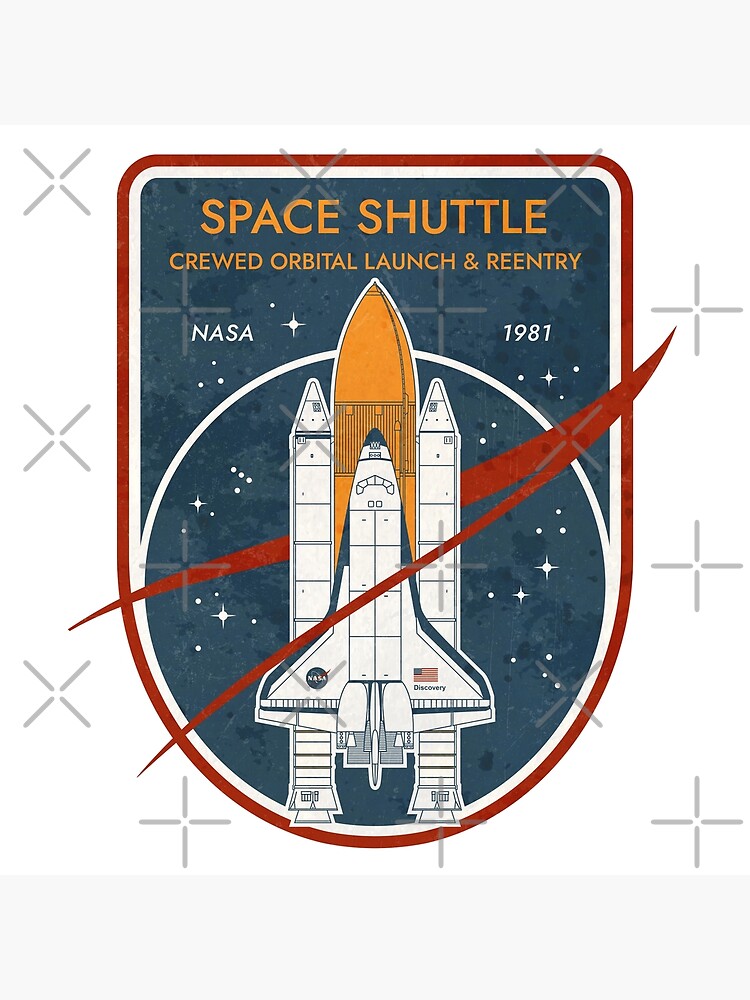This image features an intricately designed NASA patch against a white background. The patch itself is semi-rectangular with a curved bottom and a prominent red outline. Dominating the patch is a depiction of a Space Shuttle, complete with two rockets, a main body, and visible propulsion units at the base. The central rocket's upper section features a gold dome, almost touching the patch's top. Just above this dome, in elegant gold lettering, is the phrase "Space Shuttle, Crewed Orbital Launch and Reentry." The background is a dark greenish-gray, speckled with tiny white stars that evoke a night sky. To the left, beneath the gold lettering, is "NASA" in white, and to the right, the year "1981." A bold red swish arcs behind and in front of the shuttle, adding dynamic motion to the design. Furthermore, in front of the red swish, a white oval encircles the shuttle. The patch features additional design elements, including the American flag and the word "Discovery," hinting at the Space Shuttle Discovery. The entire image resembles a badge or t-shirt graphic, blending dark red, bronze-orange, yellow, and navy blue to create a vivid and compelling representation of a historic space endeavor.